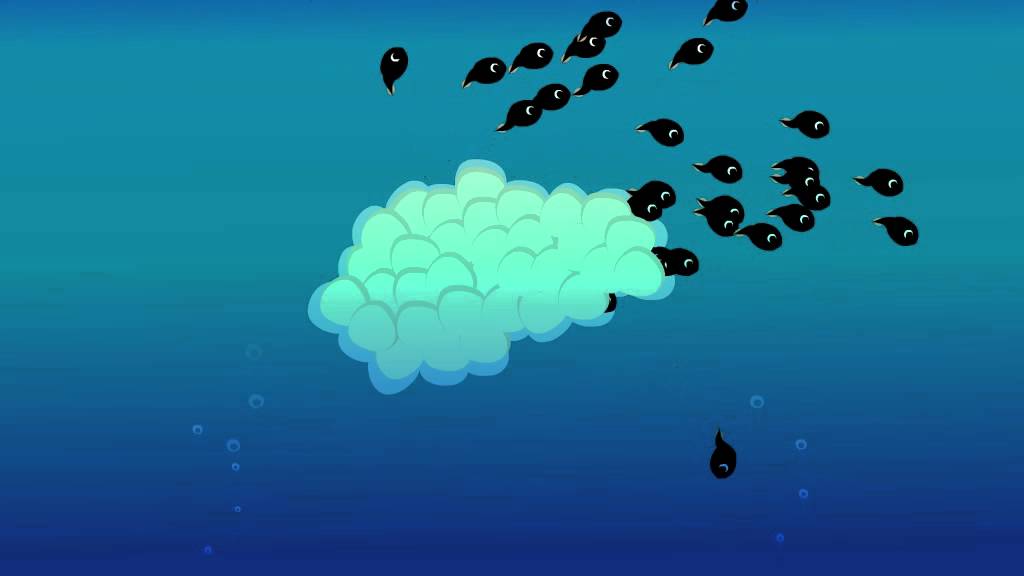The image is a detailed and stylized digital artwork depicting an underwater scene. The background transitions from a dark blue at the bottom, through aqua in the middle, and then to a lighter blue at the top, forming a gradient that gives a sense of depth. Small air bubbles are visible, rising from the bottom of the image. Dominating the center is a large, bulbous white-cloud-like structure, which likely represents a cluster of eggs. Emerging from this cluster are approximately 20 small, teardrop-shaped creatures with tiny, wiggling tails. These creatures resemble tadpoles, each featuring a simple design: an oval body tapering to a point near the tail, a single eye marked by a white crescent shape. They also have clear fins on their tails, one on the top and one on the bottom. The tadpoles are swimming in various directions; most are moving to the right, while a few swim straight up or down. The overall scene beautifully captures the early life stages of amphibians in a vibrant, animated style.